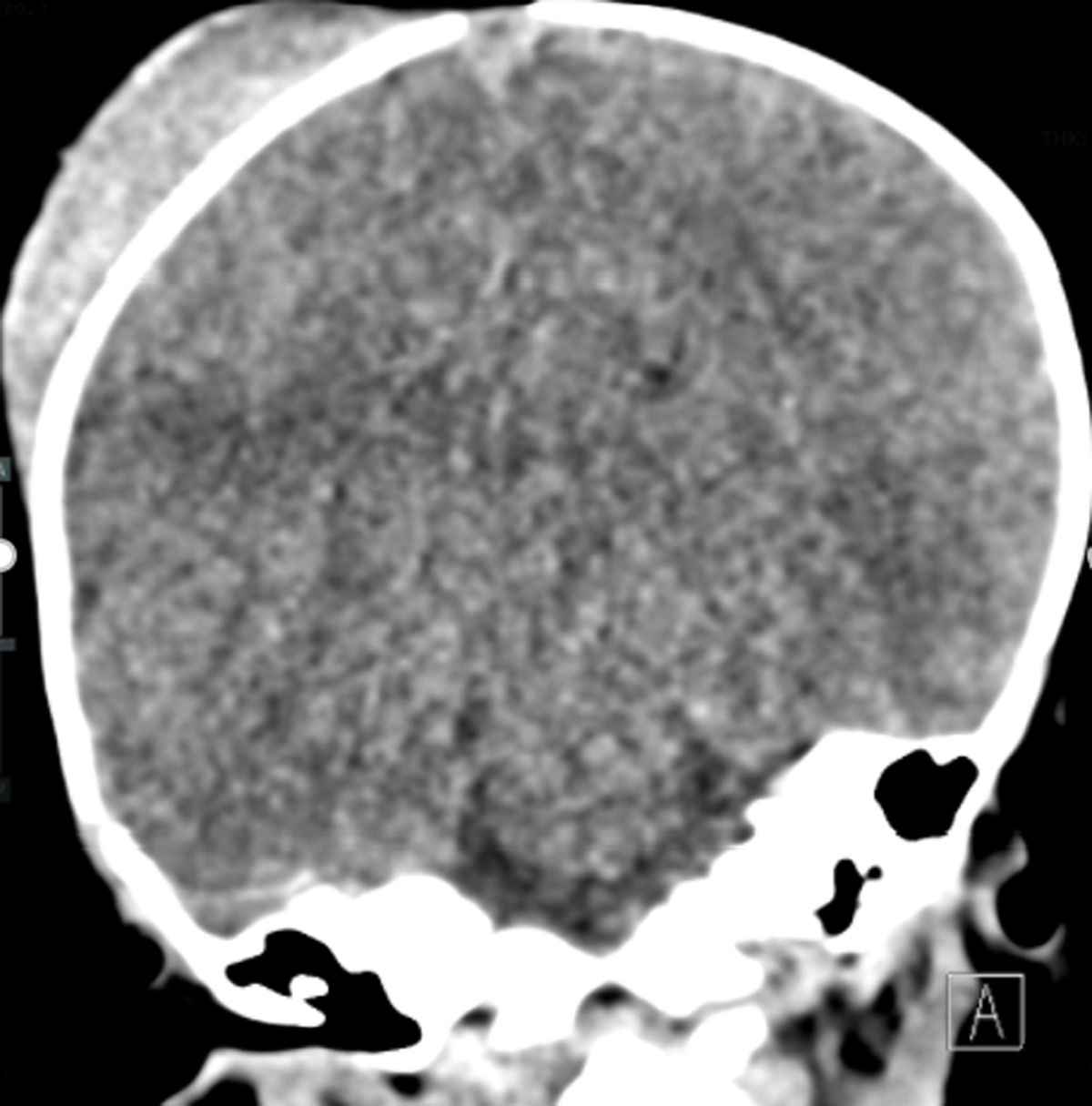This is a detailed image caption combining elements from all three descriptions:

The image is a black, white, and gray medical scan, likely an MRI or CT scan of a human brain. It is presented against a completely black background, emphasizing the circular or round shape that suggests it could be a section of a skull. The image is marked by a white outline around the perimeter, except for a small gap at the very top, which provides contrast against the gray and dark gray matter within. The interior appears somewhat staticky or pixelated, with black splotches indicating areas of less density, such as possible indentations or holes in the brain structure. A distinctive feature is a labeled box with the letter "A" located in the bottom right corner of the image, serving as a label or identifier. Despite the low resolution, the scan prominently displays the brain’s central region, dominated by gray matter, making up the majority of the image.